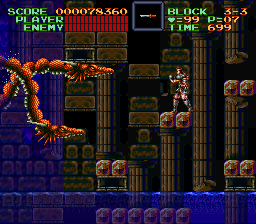The image is a captured scene from an old-school, retro video game, possibly from the 90s, potentially identified as either Rygar or Castlevania. Dominated by vibrant colors, this pixelated display shows two dragon-headed serpents on the left, distinguished by their long, snake-like bodies, green horns, and green spikes on their undersides. These dragons are suspended in the air, facing a knight character poised in green armor, with parts of his legs and face exposed. The knight, presumed to be the main character, stands on platforms constructed from two stones with a diamond in the middle.

In the background, old building columns partially submerged in blue, water-like coloring are visible, along with sections of brown bricks. The game's HUD at the top of the screen displays various details: a score of 000078360 in yellow font, health bars for player and enemy indicated by red bars, and additional game stats such as "block 3-3," "hearts 99," "P=07," and "times 699." Centered in the HUD is a depiction of a single knife, suggesting the knight’s current weapon. The overall scene blends elements of adventure and fantasy typical of iconic 90s video games.